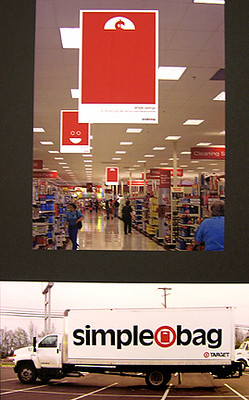This color image consists of two separate photographs arranged vertically on a large rectangular canvas. The top photograph, which occupies approximately 70% of the space and is framed with a thick, grayish-black border on three sides, depicts the bustling interior of a Target store. This image showcases various shoppers browsing through aisles filled with products. Hanging from the ceiling are prominent, rectangular banners with a white background and red shapes, including a dollar sign and a smiley face, suggesting promotional offers or discounts.

The bottom photograph, smaller in size and taking up about 30% of the overall image, features a white box truck parked in a lot and facing left. The truck's side displays the words "Simple Bag," with a red circle containing a red square serving as a logo between the two words. Additionally, the Target logo and the word "Target" are visible beneath this design. The truck has black wheels and brownish-silver rims, emphasizing its robust, utilitarian appearance.